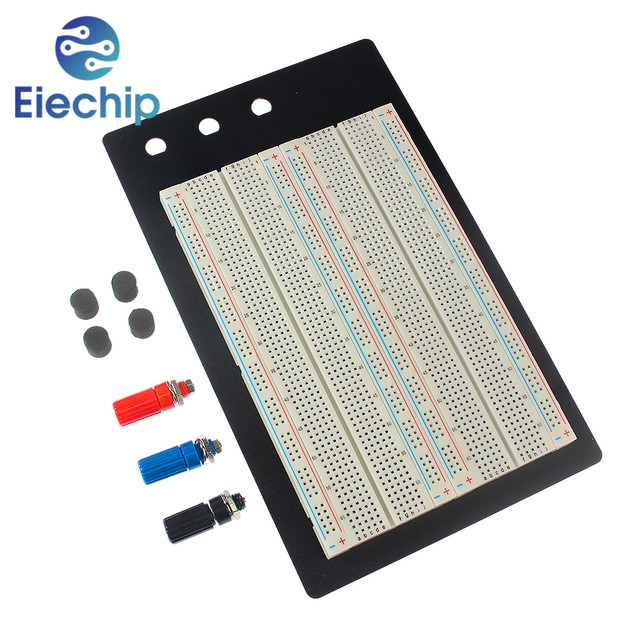The image depicts a detailed test or circuit board, prominently featuring a blue circular logo in the upper left corner that reads "EIE chip". This white circuit board is adorned with numerous rows and columns of small holes, meant for connecting electrical components without soldering. Vertical stripes of blue, red, and gray enhance the grid-like appearance of the board. Adjacent to the board on the left are a series of components: four cylindrical black caps, and three colored devices—a red one, a blue one, and a black one—that resemble audio jacks or dials. Additionally, there are small foam pieces situated nearby. The overall setup appears to be an electrical circuit connector device, ready for engineering or testing purposes.